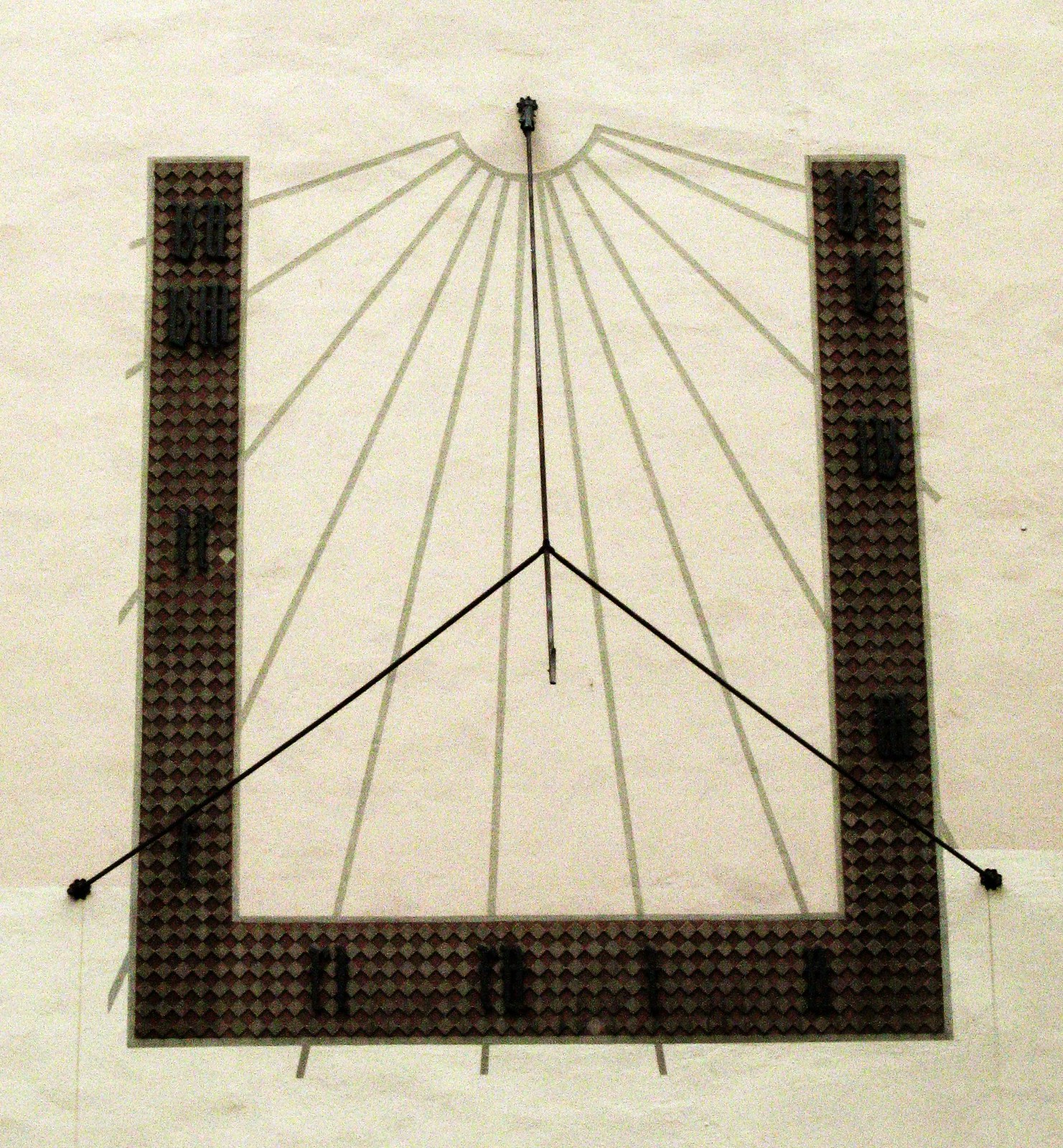The image showcases an intricate piece of art or a graphic that mimics an architectural or mechanical design, potentially inspired by a bridge structure or a sun meter. Dominating the composition is a bold, geometrical U-shape, constructed from dark, rectangular segments which exhibit an Argyle-like texture. This U forms a frame around the central features of the artwork, extending up the left side, across the bottom, and up the right side.

In the middle of this U-shape, a black triangular area bisects the space, intersecting with the bottom part of the U. Above this triangle, in the top center of the image, a central focal point emanates multiple lines, reminiscent of rays extending from a sun or the spread of measuring instruments. These lines are predominantly pale green with one prominent black line descending straight down the center.

Approximately a quarter inch from the bottom of the black central line, two additional lines extend horizontally outwards, piercing through and extending beyond the boundaries of the U-shape, adding to the complex, almost diagrammatic quality of the piece. The overall color palette features shades of black, dark brown, and pale brown, all set against a creamy, off-white parchment-like background, giving the piece a timeless, chiaroscuro effect filled with structured elegance.